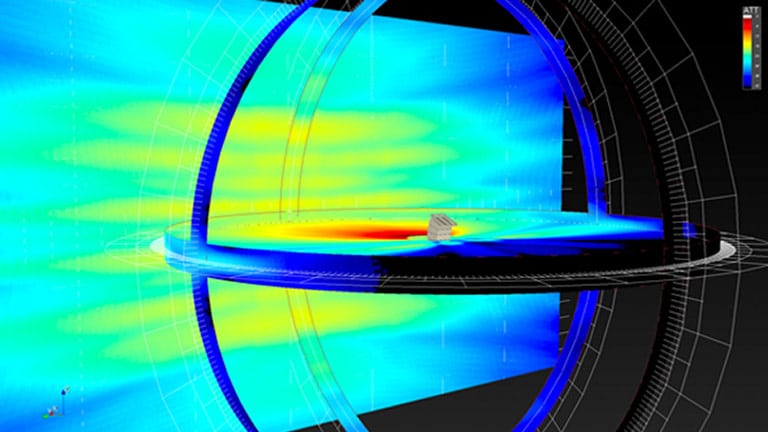This image features a computer-generated sphere-like structure composed of intersecting rings, suggesting the semblance of a globe. At the core of this intricate formation lies a circular three-dimensional plate, centering the design. This central plate is adorned with a vibrant tie-dye pattern, showcasing a spectrum of colors from red, orange, and yellow to green and blue. Situated behind this orb-like centerpiece is a large, slightly bent rectangular shape, echoing the same tie-dye color scheme of blue, yellow, and green. The right side of the image is enveloped in black darkness, punctuated with fine lines. Completing the composition, there is a small scale at the top displaying a gradient of colors ranging from red to blue, reminiscent of a rainbow.